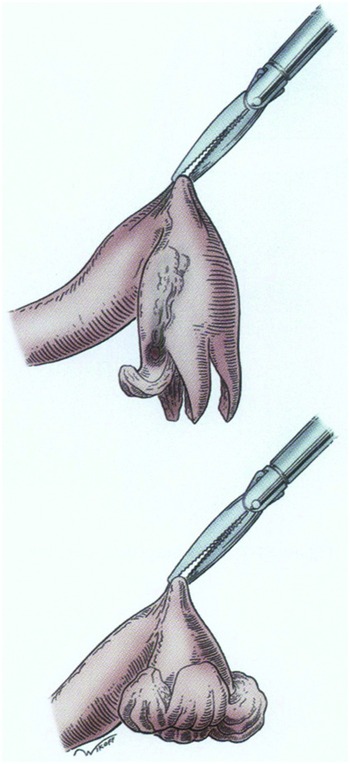The illustration features two detailed drawings against a light blue background, showcasing a metal device, likely silver forceps, holding an ambiguous natural object, possibly a flower or an animal part. The forceps have rigid teeth and grasp the object in two different positions. 

In the top illustration, the forceps pinches a pink, limb-like object that hangs down limply, displaying four petal-like extensions, one of which flips upward. The object appears to be a part of some yet unidentified entity, its pink hues contrasting with the metallic sheen of the prongs.

The bottom illustration depicts the same scene but with the pink object now with its petal-like extensions curled up tightly towards its body, resembling a clenched fist. The artistry employs hatching techniques to create shading, maintaining a highly detailed yet non-photorealistic style. On the lower left corner of the image, a signature in black can be observed, indicating the artist's mark.